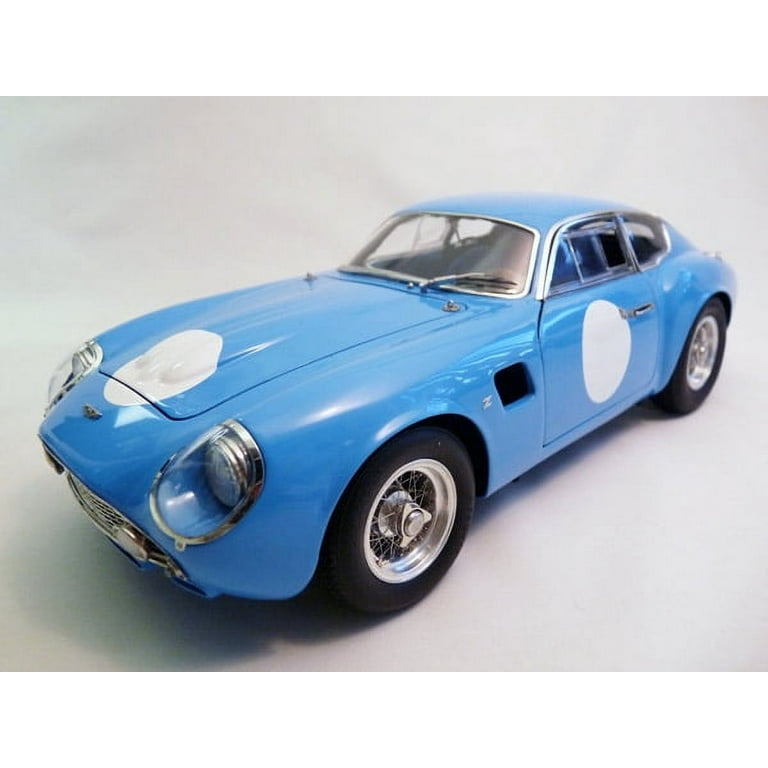This image features a light blue, vintage Jaguar XKE, or a similar old sports car model, with prominent chrome accents. The car, which resembles a blunted shark or even a bug-like shape, is facing the bottom left corner of the frame. The vehicle is detailed with white circular decals, one on the hood near the front bumper and another on the driver's side door. The car sports round, slightly sunken headlights encased in chrome, and a chrome front grille beneath them. The windows on the doors and the small rear window are also bordered with chrome, as are the windshield edges and the door handles. The chrome extends to the black tires' rims, highlighting the car's polished look. The car casts a shadow against an off-white background, further emphasizing its three-dimensional form. A single windshield wiper, which is chrome and black, arcs from the driver's side towards the passenger's side. Additionally, an air intake or exhaust opening is visible on the back of the driver's side fender, suggesting intricate design details. Despite the image's realistic appearance, it could be a highly detailed model car.